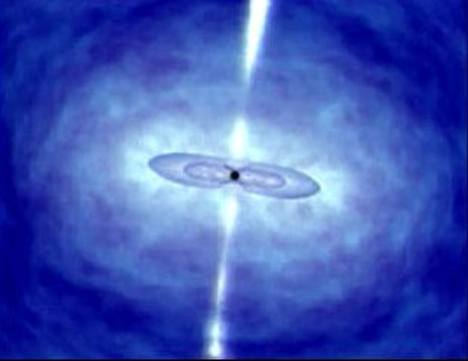The image, potentially depicting a science-themed or abstract scene, presents a striking composition. It features a rich blue background that darkens towards the edges and lightens towards the center, creating a vivid contrast. Central to the image is a small black dot, from which emerges a delicate, slightly angled oval extending horizontally from left to right. Within this larger oval, a smaller inner oval is visible due to a subtle light delineation. Surrounding the central elements, wispy white formations give the appearance of ethereal clouds. Additionally, a white vertical streak runs from the bottom to the top of the image, intersecting the central black dot and adding to the captivating visual effect. This central streak gives the impression of a dynamic force, like light or energy, cutting through the serene blue backdrop. The intricate details and interplay of colors suggest themes of space or abstract art, leaving viewers to ponder the exact nature of the scene.